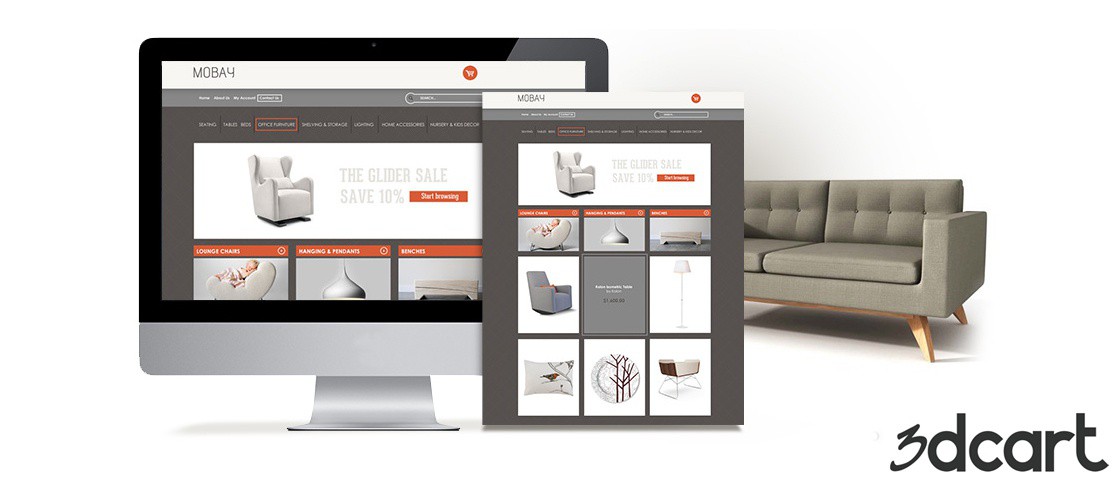A detailed and cleaned-up caption for the image could be:

"In this screenshot, the company name '3DCART' is prominently displayed in the lower right corner with the number '3' in a larger font and 'D-C-A-R-T' in smaller letters. On the left side of the image, there's a computerized interface, while the right side shows a webpage. The webpage screenshot prominently features the top section of the website, showcasing a modern furniture setup. This includes a stylish mix of contemporary chairs, couches, lamps, pillows, and other decor items. Even though the text on the webpage is somewhat difficult to read, it appears to advertise a promotion with light gold text reading something like 'Glider Sale - Save 10%.' In the center background of the monitor display, there's a partial view of a modern brownish-gray couch with light brown wooden legs and a supportive board, though part of it is obscured by the on-screen elements."